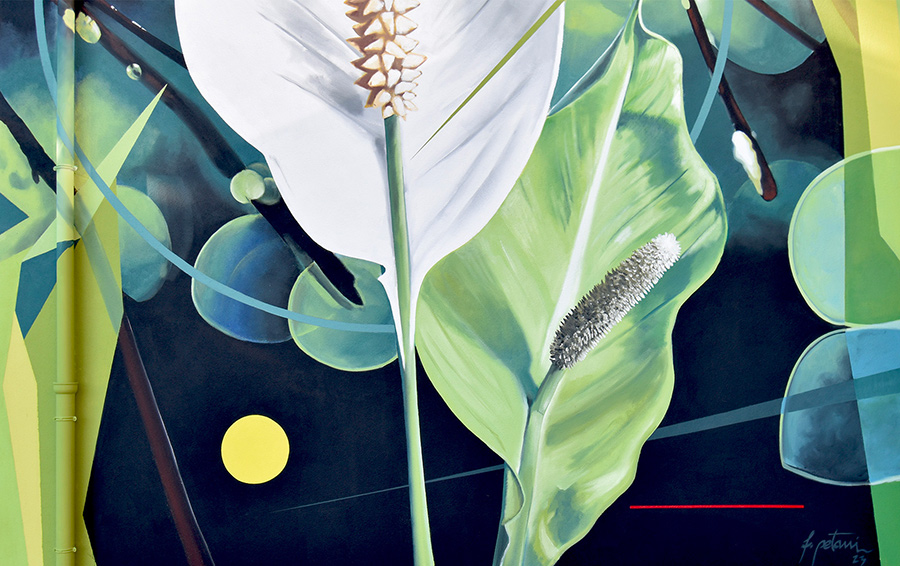The image depicts a vibrant, modern abstract painting with a mix of surreal elements. Central to the composition is a white leaf with a green stem, partially overtaken by a large, wavy leaf that has a thistle-like fuzzy center. Surrounding this are various shapes and elements: green, white, and blue leaves, a striking yellow dot against a solid blue background, and round shapes set against black. Yellow lines cascade down the sides, while black sticks resembling dogwood branches, adorned with white fuzzy details, add a dynamic touch. The painting also features a horizontal red line in the bottom right corner, alongside a signature by the artist. The overall scene is brightly illuminated, bringing clarity to the intricate details and contemporary style of the artwork.